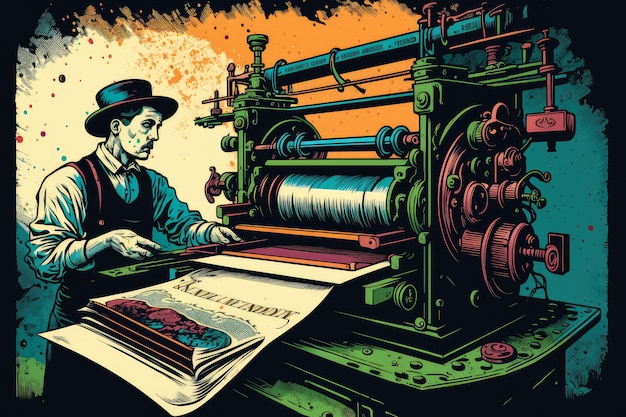This vibrant and detailed color illustration depicts a man operating a complex 19th-century printing press. The man, a white male and printer, is dressed in a black bowler hat, a white button-up long-sleeved shirt, and a black apron. He stands to the left of the large, intricate machine, which dominates the foreground. The press itself is an elaborate assembly of green, blue, and red components, with gears and cranks painted a striking pinkish-purple and red. The roller at the center of the machine is actively printing, producing pages that exhibit a range of colors including purplish-blue and red. The finished newspaper pages emerge from the press, showcasing detailed images and text.

The background is a colorful mosaic of blue, orange, and white, with areas spattered in paint, contributing to the lively atmosphere of the scene. Notably, there are tan, turquoise, and orange ink splotches dotting the black backdrop, enhancing the artistic and somewhat chaotic setting. The lower part of the machine is primarily dark green, with blue lateral posts situated at the top. This intricate setup brilliantly captures the essence of an old-world print shop in full swing.